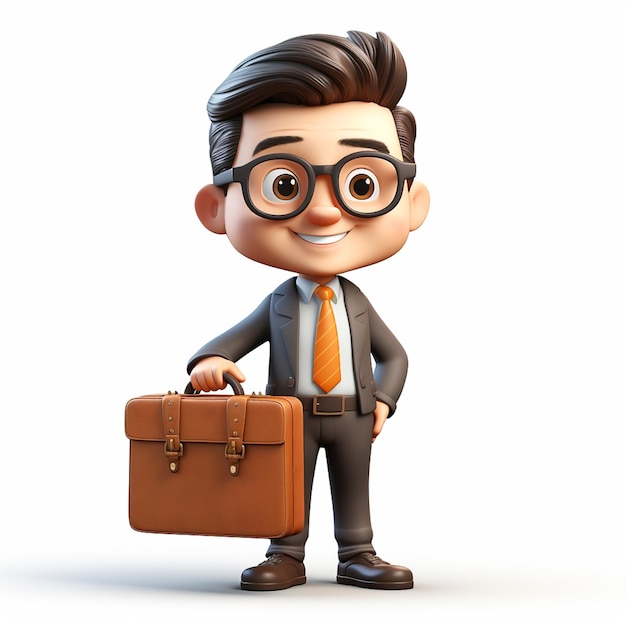This is a brightly-colored, computer-generated image in a very 3D, bubbly animation style, featuring a short, white cartoon man with a disproportionately large head. He has short brown hair, styled traditionally to one side, with a plasticky sheen under the light. His expressive face includes big black round glasses, raised eyebrows, brown eyes, a button nose, and a wide, enthusiastic smile. He wears a well-fitted gray suit paired with an orange tie adorned with white stripes, a crisp white collared shirt, and a black belt with a gold buckle. Completing his outfit are brown dress shoes. In his right hand, he holds a light brown leather briefcase, detailed with two buckled straps and a black handle, completing his professional appearance.